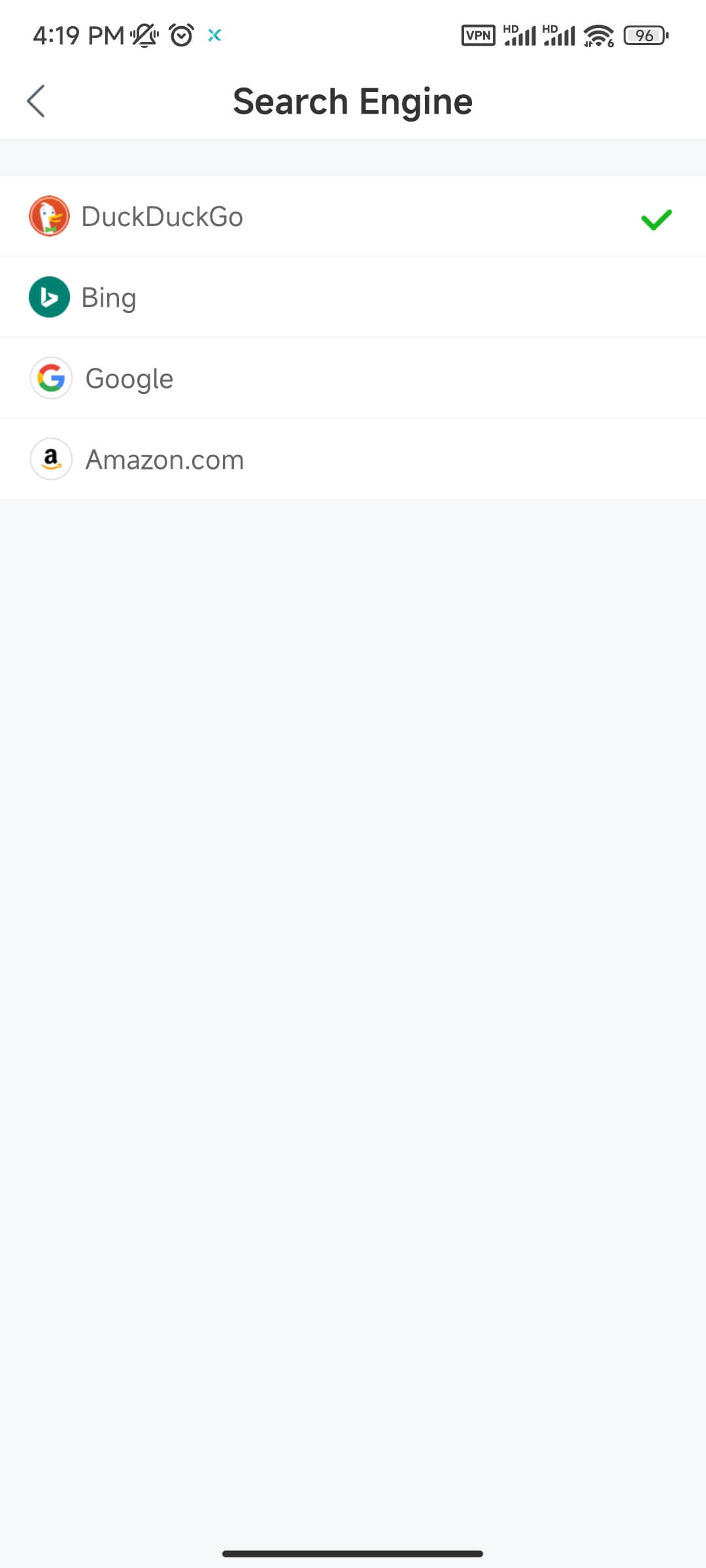This is a detailed screenshot of the search engine settings tab on a mobile phone. At the top of the screenshot, the heading "Search Engine" is displayed prominently in bold black font. Below this heading, there is a compact vertical list of browser options. The list includes DuckDuckGo, Google, and Amazon, with DuckDuckGo selected as the default search engine. The background of the screenshot is a muted grey color, and the image is in a mobile landscape orientation. 

The top bar of the phone is partially visible, featuring various status icons. On the far left, the current time is displayed, accompanied by icons for sound off and an active alarm. On the far right, there are icons indicating an active VPN connection, signal strength, and battery level. The bottom portion of the screenshot is cropped out, omitting the phone's icon dock.